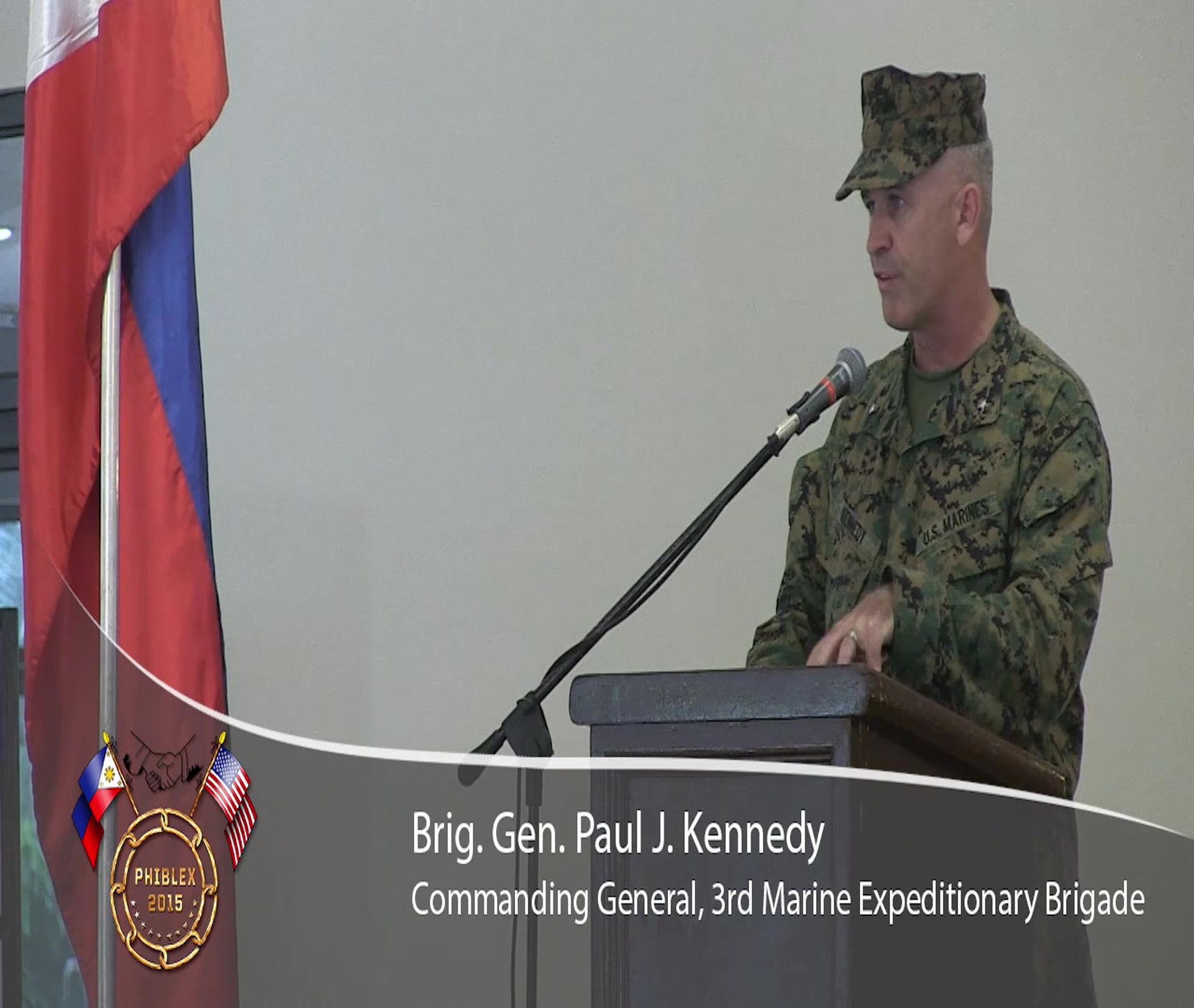The image features Brigadier General Paul J. Kennedy, Commanding General of the 3rd Marine Expeditionary Brigade, delivering a speech at a wooden podium. He is dressed in full digital camouflage fatigues, including a camouflage hat, indicating his affiliation with the U.S. Marines. He is an older, Caucasian man, wearing a wedding ring, and appears to be mid-speech, with a serious expression as he looks slightly to the left. A microphone is positioned near his face, attached to a stand on the left side of the podium. The backdrop is a plain white wall, and to the right, a red, white, and blue flag is visible. At the bottom of the image, there is white text on a semi-transparent gray background that reads "Brigadier General Paul J. Kennedy, Commanding General, 3rd Marine Expeditionary Brigade." To the left of this text is an emblem with crossed flags: one depicting a red, white, and blue flag with a yellow sun, and the other the American flag, labeled "PHIBLEX 2015."